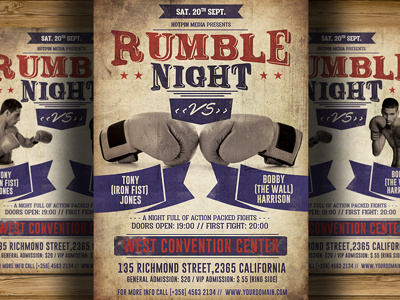This promotional poster for a boxing match prominently displays a blue banner with white lettering in the center, announcing "Saturday 20th September." Below that, it reads "Horton Media Presents" followed by "Rumble Night" in red and "Versus" in blue. The focal point of the poster features two white boxing gloves touching each other. Under the left glove, the name "Tony 'Ironfish' Jones" is displayed, while under the right glove, it says "Bobby 'The Wall' Harrison." Further details include "A Night Full of Action-Packed Fights," with doors opening at 19:00 and the first fight starting at 20:00, at the West Convention Center, located at 135 Richmond Street, 2365 California. Ticket prices are listed as general admission for $20 and VIP ringside admission for $55. For more information, a phone number (356-456-32134) and a website (www.yoursomething.com) are provided. The design features pictures of Tony and Bobby on the left and right sides, respectively, with a cream, brown, and navy blue color scheme, giving it a vintage, newspaper-like aesthetic.